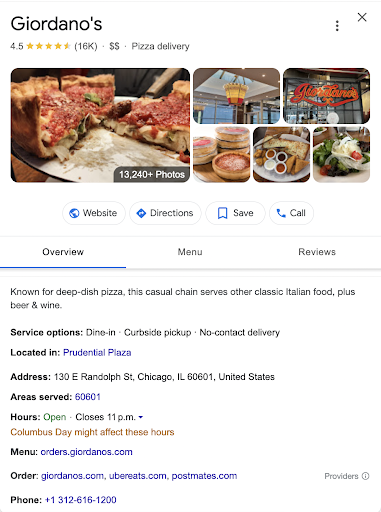Giordano's—an acclaimed Italian restaurant located at 130 East Randolph Street, Prudential Plaza, Chicago, Illinois, 60601—is renowned for its deep-dish pizza and holds a stellar 4.5 out of 5-star rating based on 16,000 reviews. Their offerings include a diverse array of classic Italian dishes, such as various pizzas, salads, and more. The establishment provides multiple service options including dine-in, curbside pickup, and no-contact delivery.

Prominently featured on search results, Giordano's presents images showcasing their inviting restaurant ambiance and delectable food items. Below these visuals, patrons can find convenient links for their website, directions, and contact options, including a button to call the restaurant directly. The search result also highlights the restaurant’s operating hours, with closing time at 11 p.m., though holiday schedules like Columbus Day may impact these times. 

Further, there are links available for online ordering through websites like order.giordanos.com, UberEats, and Postmates. Giordano's specializes in creating a memorable dining experience with a hearty menu complemented by a selection of beers and wines.